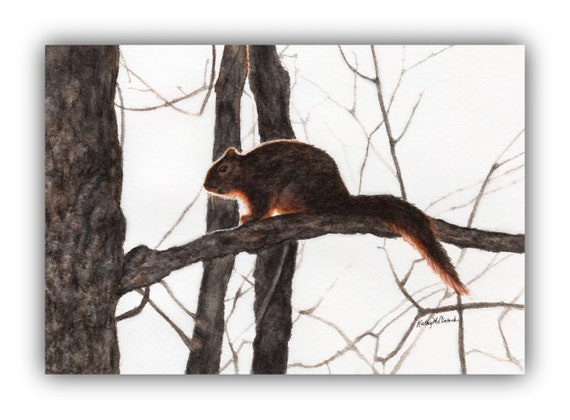In this photograph, a squirrel is perched on a branch extending from the left side of the image, appearing against a backdrop of a stark white sky, indicative of a winter scene. The squirrel, coated in shades of brown with hints of red, tan, and a touch of black fur, is captured in daylight with its eyes open, presenting a sharp contrast against the bright background. The branch it sits on, along with surrounding smaller branches, showcases a mix of brown, whitish, and tan hues, adding to the textured environment. Additional branches and tree trunks can be seen behind the squirrel, weaving intricate patterns throughout the photograph. These elements contribute to a shadow effect across the scene. In the lower right corner, a faint, albeit discernible, signature—potentially reading "Kathy Willanick"—is present, marking the creator of this serene, detailed outdoor capture.